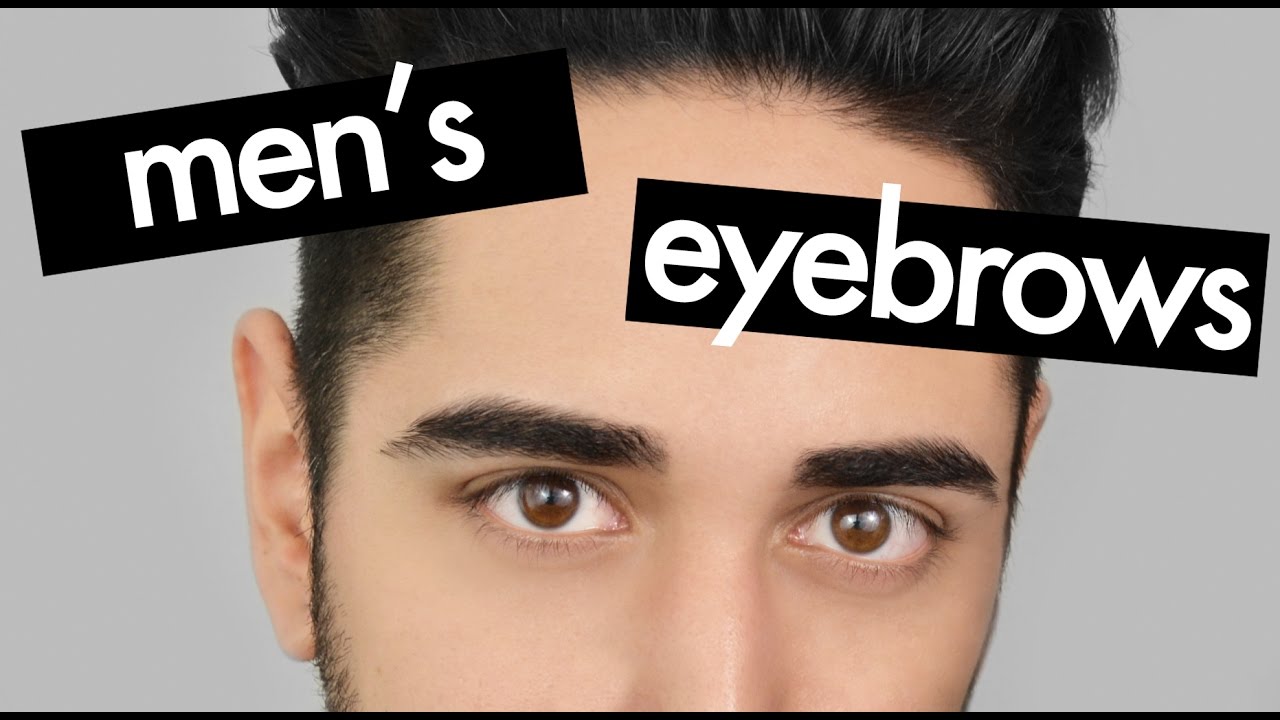This color photograph captures a young man in his early twenties from just below the bridge of his nose upward, against a light gray background. His smooth, clean-looking skin accentuates his striking features, which include bright brown eyes and neatly groomed, thick black eyebrows. His jet-black hair is styled with a product, combed back with fullness on top and tightly shaven sides, complemented by visible long sideburns. The image includes minimalistic text overlaid in white within two black rectangular boxes; one near the top left corner that says "men's" and another towards the right that says "eyebrows." The tip of one ear is visible, while the other ear can be seen more fully. Thin black lines frame the photograph from the top and bottom, adding to the clean and focused presentation.